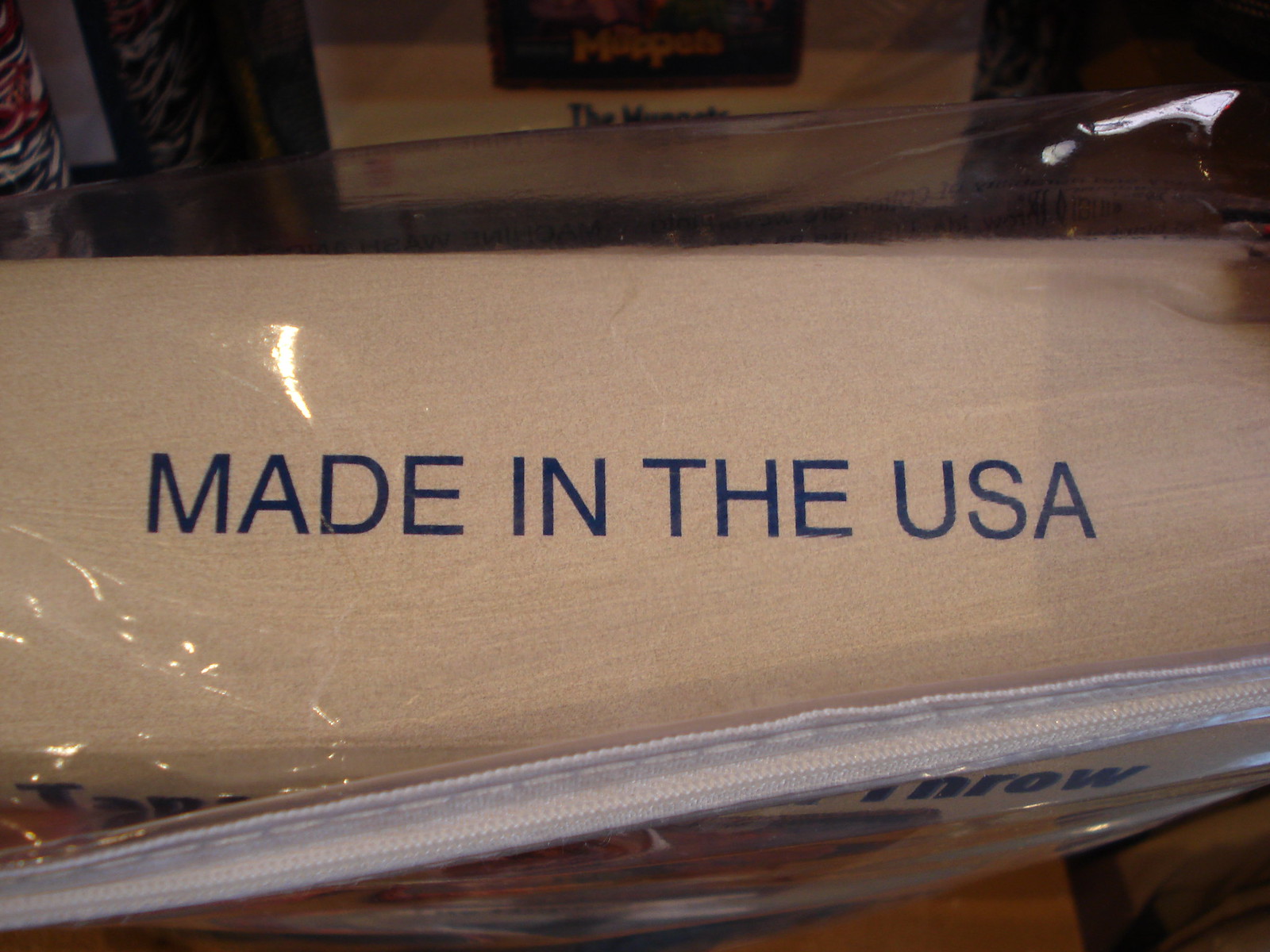In this detailed color photograph, we are looking down at a cardboard box encased in a zippered plastic bag, reminiscent of the type used for storing blankets. The box features dark blue text reading "Made in the USA" prominently displayed on its front side. Covering the front of the plastic bag, we observe a white design with the word "Throw" in dark blue text, though the letter "T" is partially obscured by the white zipper, which runs from the bottom left corner up towards the right-hand side. Below this setup, a light brown table is visible at the bottom edge of the photo. In the bottom right corner, there is a glimpse of a green tarp on the ground. In the background, another cardboard box can be seen with orange text and dark blue text beneath it, partially obscured by lighting. Additionally, on the left side of the image, a pair of very tall boots featuring red, white, and black patterns are visibly positioned, adding to the overall complexity of the scene.